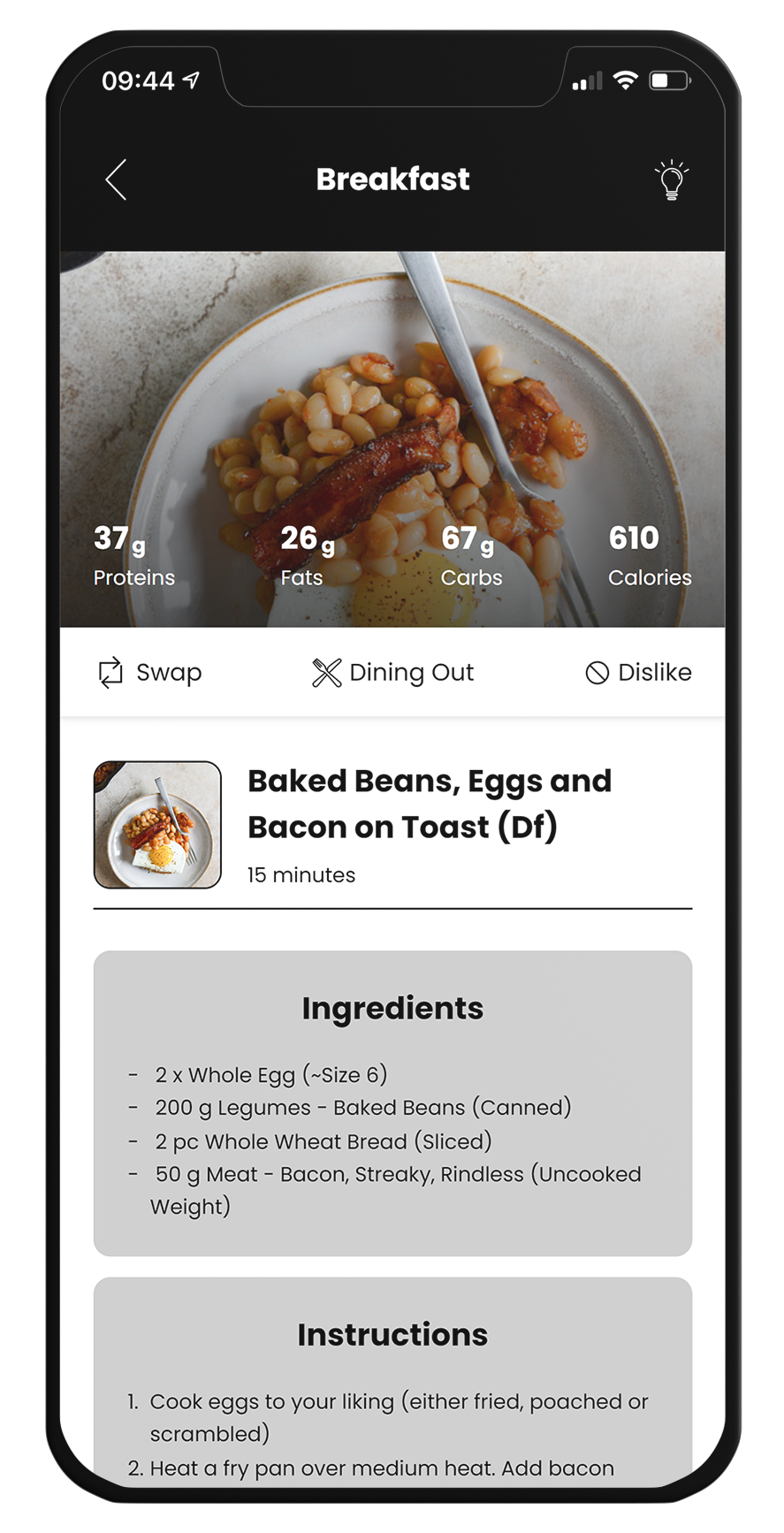**Detailed Caption:**

The image displayed on the phone screen is a breakfast recipe. At the top of the screen, the time is indicated as 9:44 AM. To the right of the time, there's an upward-pointing arrow, followed by some black space, and then two bars indicating a weak Wi-Fi signal. Next to the Wi-Fi icon is a half-full battery icon.

Below this top bar, a lighter-colored bar features a left-pointing arrow on the left side, the word "Breakfast" (capitalized) centered, and a lightbulb icon on the right side.

The main image shows a hearty breakfast meal consisting of beans and bacon on a plate, accompanied by a fork. Nutritional information is provided: 37 grams of protein, 26 grams of fat, 67 grams of carbs, and a total of 610 calories.

The following section of the screen has a white background. It starts with three icons: a swap icon, a dining out icon (depicted with a knife and fork), and a dislike icon.

The next section is slightly grayed out and has an image of baked beans, eggs, and bacon on toast, labeled with "DF" (likely indicating Dairy-Free) and the preparation time of 15 minutes.

Finally, the last sections provide details on the ingredients needed and the cooking instructions.